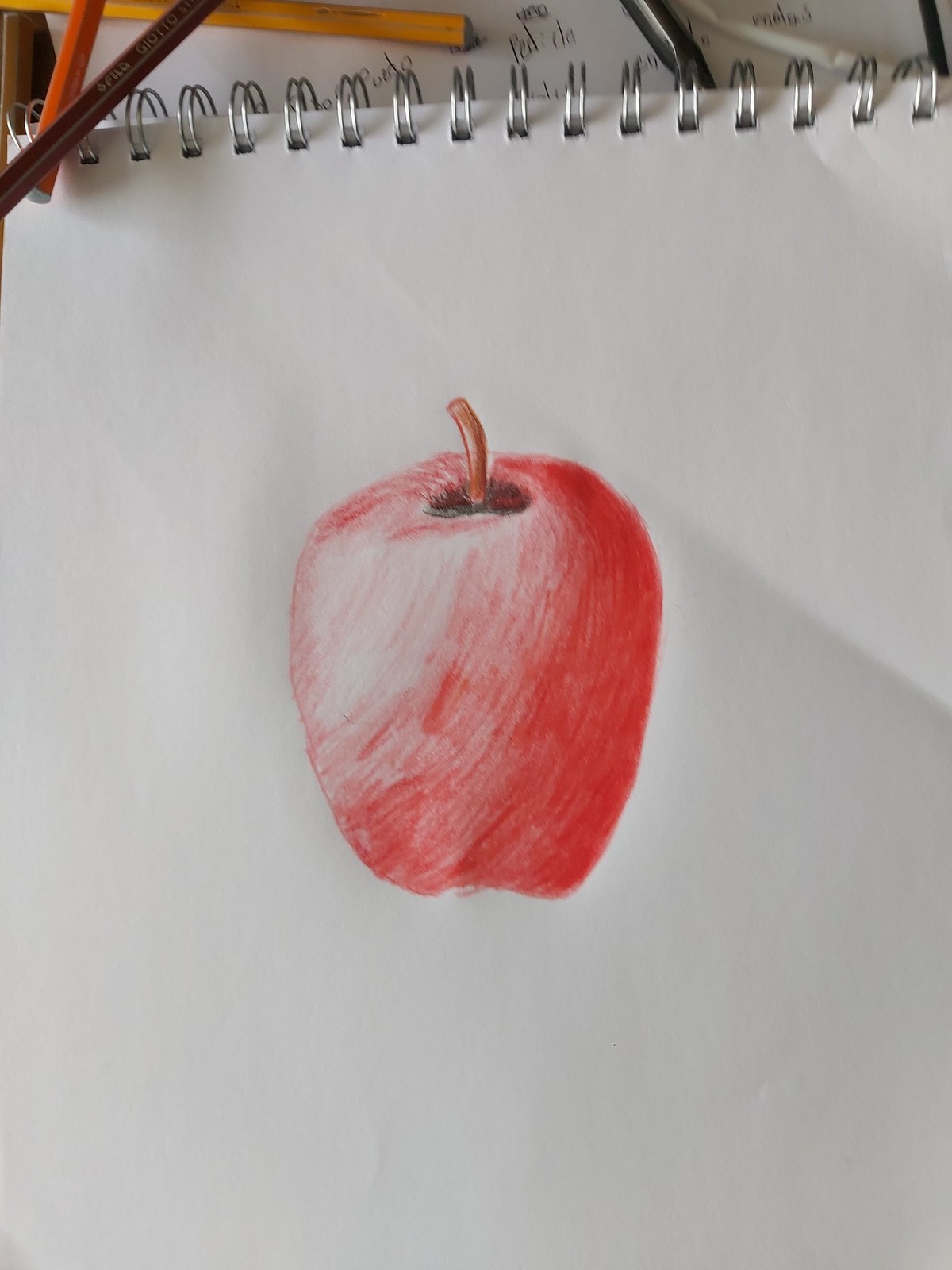The image captures a silver ring-bound drawing pad with white paper, positioned with the binder section at the top. In the upper left corner, two partially visible pencils—one maroon and the other orange—are crossed. At the center of the pad, an intricately drawn red apple takes focus, complete with a light reflection depicted on its left side. The apple features a small, brown stem, surrounded by subtle black shading to indicate shadow. The light source emanates from the right side of the image, casting a soft shadow from the top of the apple down to the lower left corner of the pad, adding depth and realism to the drawing.